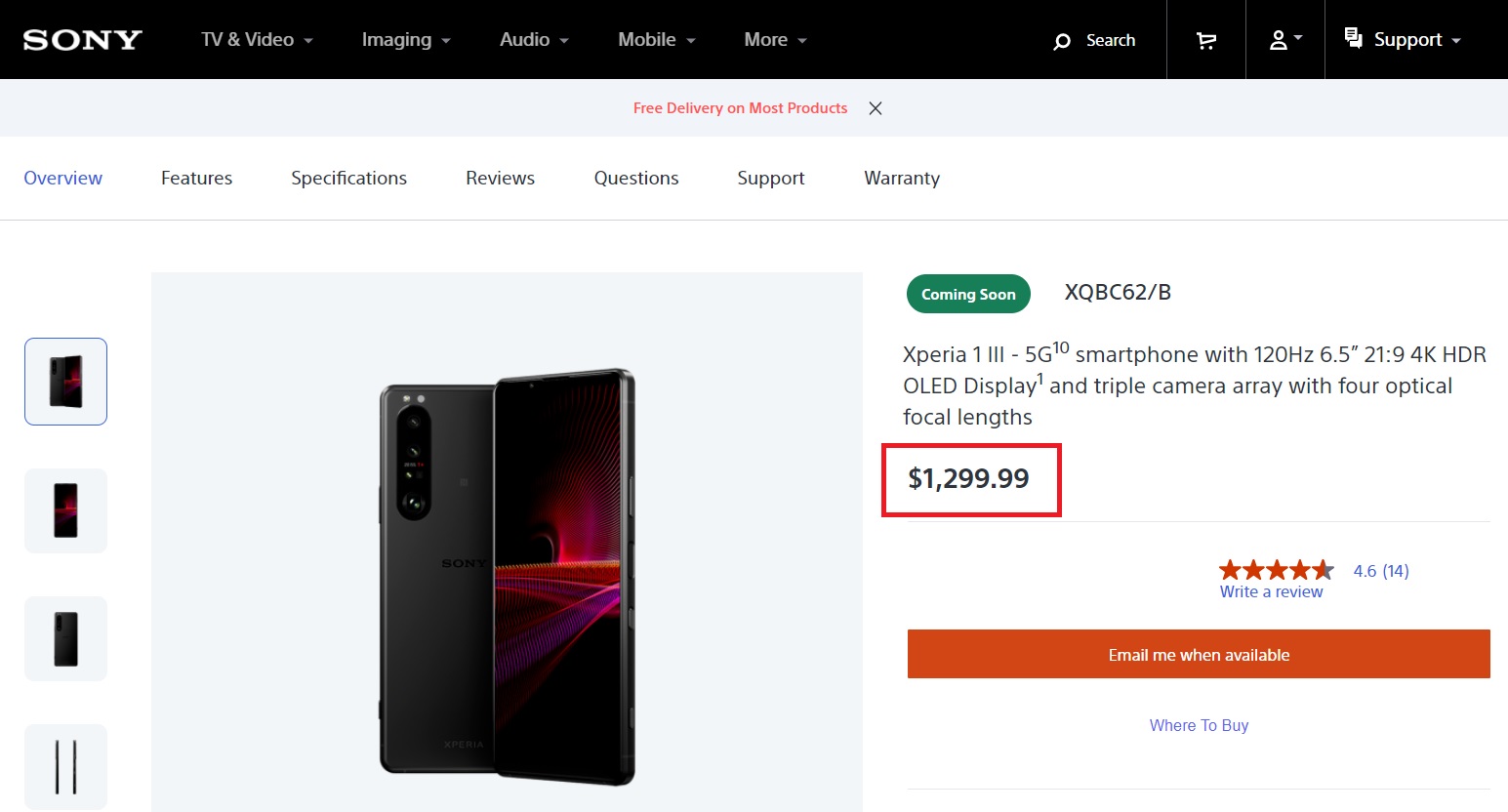**Detailed Caption:**

This image is a computer screenshot from Sony's official website. Positioned in the top left corner, the Sony logo is displayed within a black rectangular box. Adjacent to it, the navigation bar includes links titled "TV & Video," "Imaging," "Audio," "Mobile," "More," a search icon, a shopping cart icon, a user profile icon, and a support icon. A prominent message, "Free delivery on most products," is highlighted in red text.

Below the header, there are tabs labeled "Overview," "Features," "Specifications," "Reviews," "Questions," "Support," and "Warranty," offering in-depth information about the product. The featured product is identified as the Xperia 1 III-510 smartphone, boasting a 120 Hz, 6.5-inch, 21:9 4K HDR OLED display, and a sophisticated triple camera array with four optical focal lengths.

The price of the Xperia 1 III-510 is prominently displayed as $1,299.99 within a red-bordered box. Additionally, the product has garnered a rating of 4.6 stars, colored in red. An orange box containing the text "Email me when available" is also visible, indicating that the product may be out of stock. 

This comprehensive presentation provides potential buyers with detailed information and options for further engagement with the product.